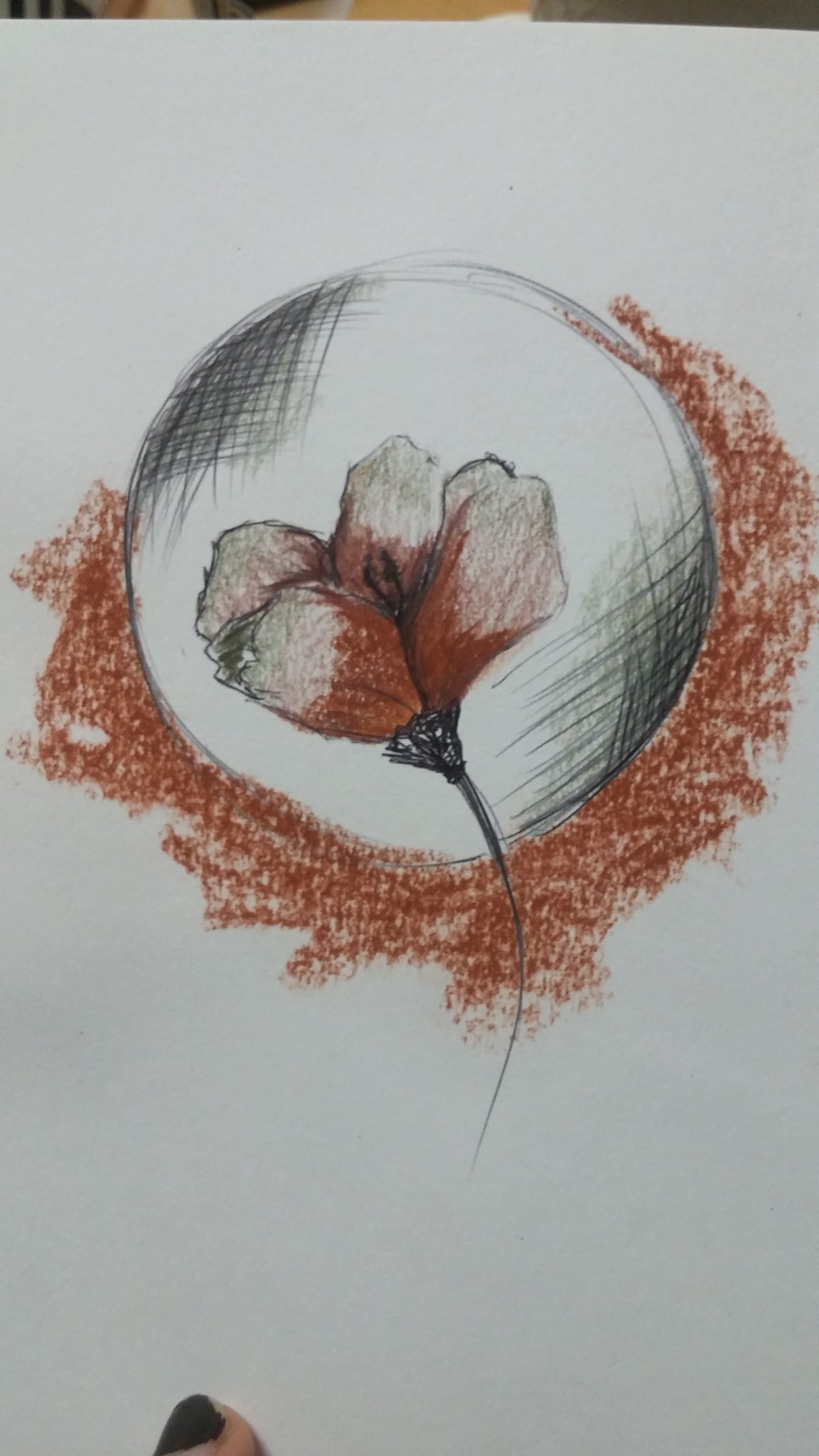The image features a drawing on off-white paper held by a person's fingertip, which is adorned with chipped black nail polish. Central to the illustration is a white sphere, or orb, shaded with intricate cross-hatching in gray and black tones at the top left and bottom right, creating a three-dimensional effect. Enveloping this orb, there's a diffuse cloud of rust to pinkish-red pastel, adding depth to the scene. Emerging from the bottom, a delicate flower stem—thicker at the base and tapering to a fine line—supports a striking flower with five segments. Each petal of the flower transitions from a dark brownish-red center to pale, grayed edges, meticulously detailed with pencil shading.